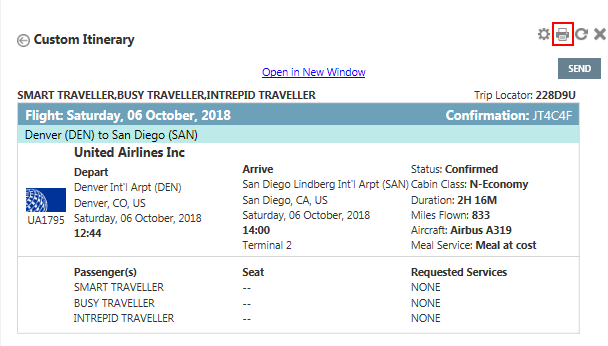Here is a detailed and clean caption for the image:

---

The webpage displays a custom itinerary interface, seemingly floating in a new window over the main screen. On the left side, the detailed itinerary information is presented, while on the right side, there are options for settings, printing, refreshing, and closing the window. Specifically, the print button is highlighted with a red box around it. 

The itinerary is titled "Smart Traveler, Busy Traveler, Intrepid Traveler," and provides the following details:

- **Trip Locator:** 228D9U
- **Flight Information:**
  - Airline: United Airlines
  - Date: Saturday, October 6, 2018
  - Route: Denver to San Diego
  - Departure: Denver International Airport (DEN), Denver, Colorado, USA at 12:44 PM
  - Arrival: San Diego International Airport (SAN), San Diego, California, USA at 2:00 PM
  - Terminal: 2
  - Status: Confirmed
  - Class: Economy (N)
  - Duration: 2 hours and 16 minutes
  - Distance: 833 miles
  - Aircraft: Airbus A319
  - Meal Service: Meal available for purchase

Passenger information is listed under "Smart Traveler," "Busy Traveler," and "Intrepid Traveler," but no seat requests or selections have been made.

---

This comprehensive caption provides a clear and detailed description of the image.